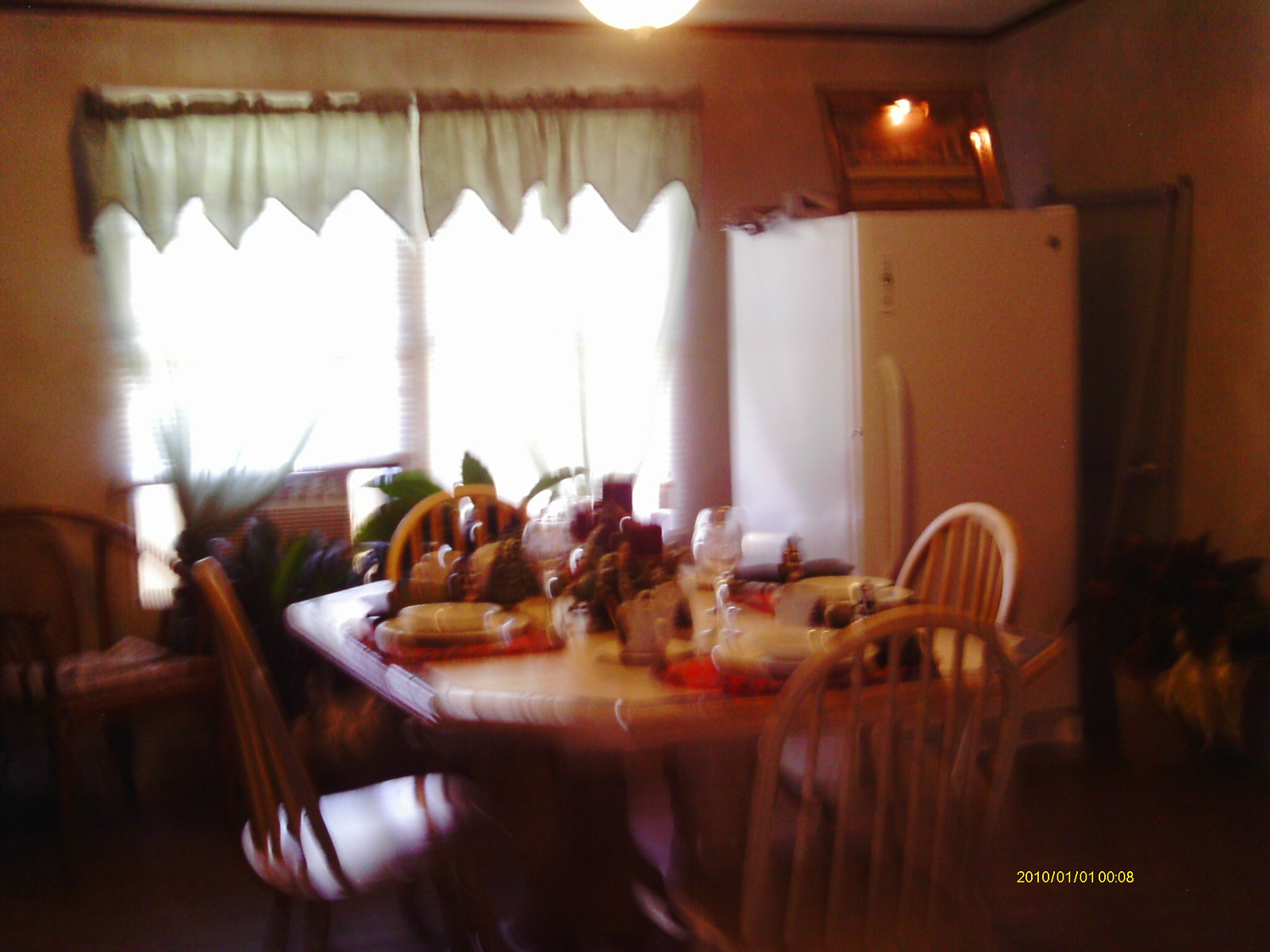This slightly out-of-focus photograph captures a cozy kitchen and dining area from a residence, timestamped January 1, 2010, at around 00:08. Central to the image is an oval-shaped brown wooden table surrounded by four wooden chairs with curved backs. Each place at the table is set with plates on red placemats, accompanied by glasses that resemble wine glasses. The table also appears to have a candle centerpiece. To the right of the table, a large white refrigerator can be seen, with some objects on top, including what seems to be a portrait of The Last Supper. The back of the kitchen is dominated by two large windows that extend from near the ceiling down to the floor, adorned with Venetian blinds. The blinds are complemented by a white fabric valance accented with a red border and a zigzag hem. A chair is placed in the left corner of the kitchen, which seems to be around 15 square feet in size. The overall color palette of the room includes browns, whites, and hints of green, possibly from a plant in view.